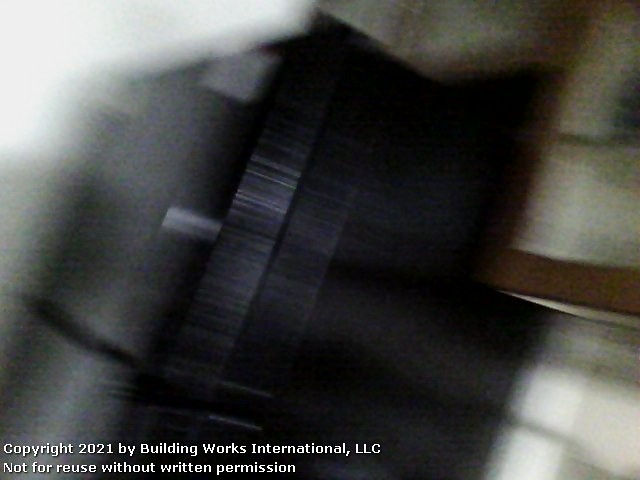The image presents a blurry scene taken indoors, likely in a kitchen area, marked by indistinct details and an unclear overall composition. Central to the image is a black refrigerator, framed by cabinetry that has a brown-like texture on the rims. The refrigerator is set within an indention specifically designed to fit its shape. The surrounding scene includes what appears to be wooden elements, possibly shelves or a door frame, and a black floor. Additional elements such as flannel shirts in brown and gray colors seemingly draped in the background add to the indistinct clutter. In the bottom left corner, the image bears a copyright mark from 2021, attributed to Building Works International, LLC, indicating it is not for reuse without written permission.